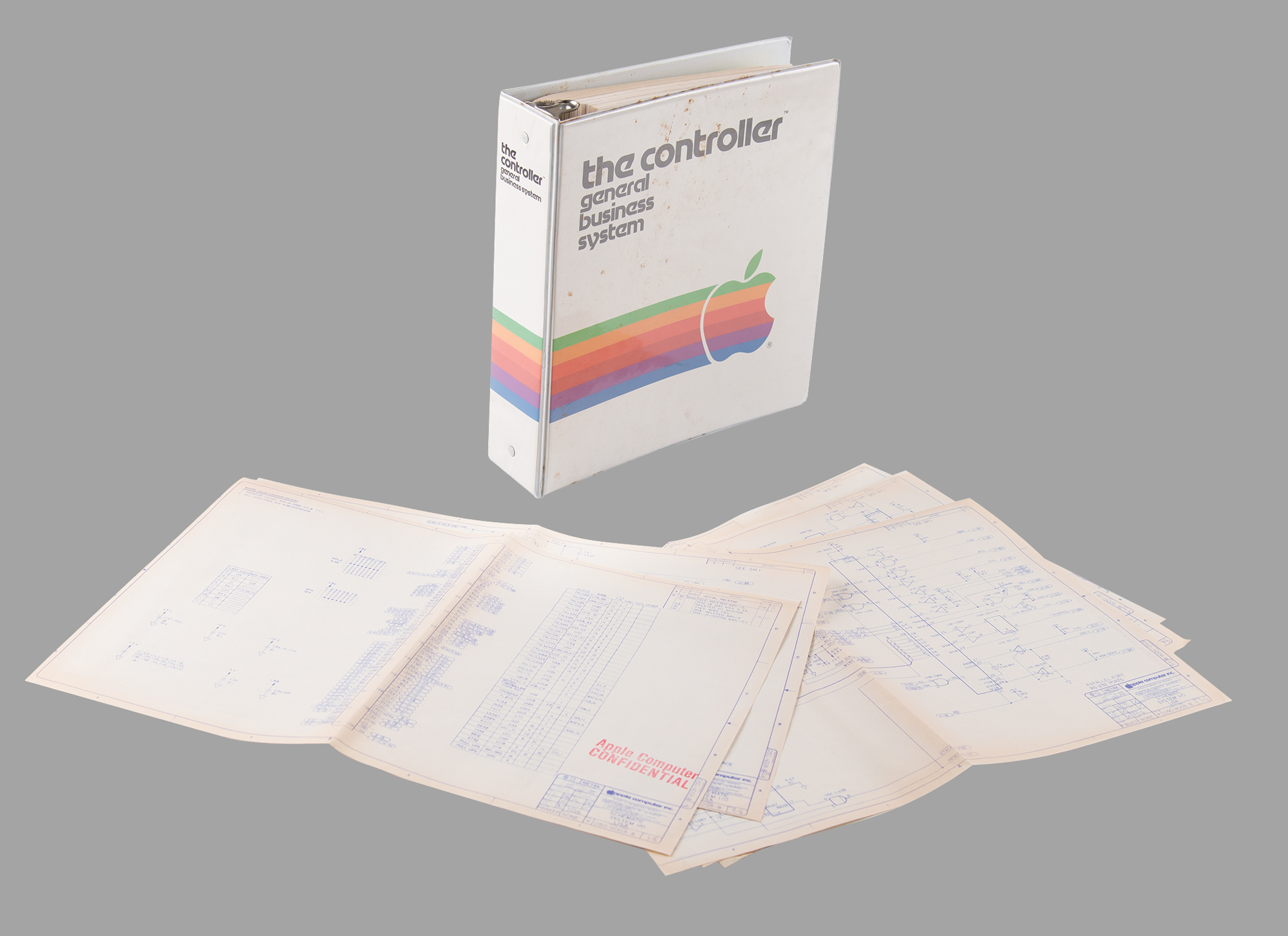This image showcases a vintage Apple product manual titled "The Controller, General Business Systems." The manual, which appears to be a ring binder folder, is presented standing on its edge and tilting slightly to the left. The front cover and spine of the binder feature the title "The Controller, General Business Systems," along with Apple's iconic rainbow logo—an apple with a bite taken out on the right side and a small leaf on top.

In front of the binder, scattered on a matte grey background, are multiple technical sheets embossed with blue schematics, diagrams, tables, and numbers. One of the prominent sheets bears the label "Apple Computer Confidential" in red text. These papers appear highly technical, likely containing detailed repair diagrams, software instructions, and other information useful for a systems administrator. The overall setup suggests that this manual and the accompanying documents were vital resources for managing and troubleshooting Apple computing systems in the past.